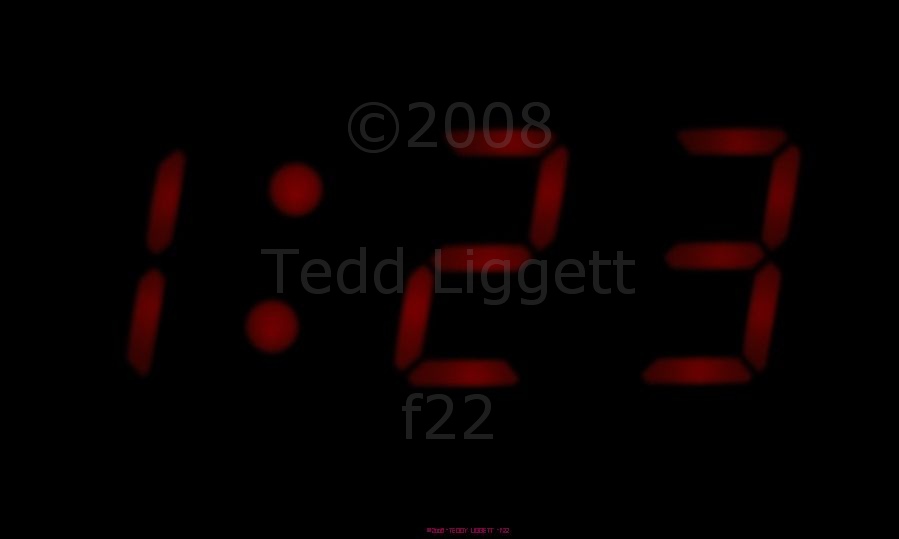A close-up view of a slightly blurry digital clock display with a black background. The time reads "1:22" in an old-style digital format where each of the seven-segment displays for the numbers 1, 2, and 3 are clearly visible. The image also features a semi-transparent watermark in a pale color that is somewhat difficult to read. The watermark is split into three lines: the top line states "Copyright 2008," the middle line reads "TEDD Liggett," and the bottom line indicates "F-22."